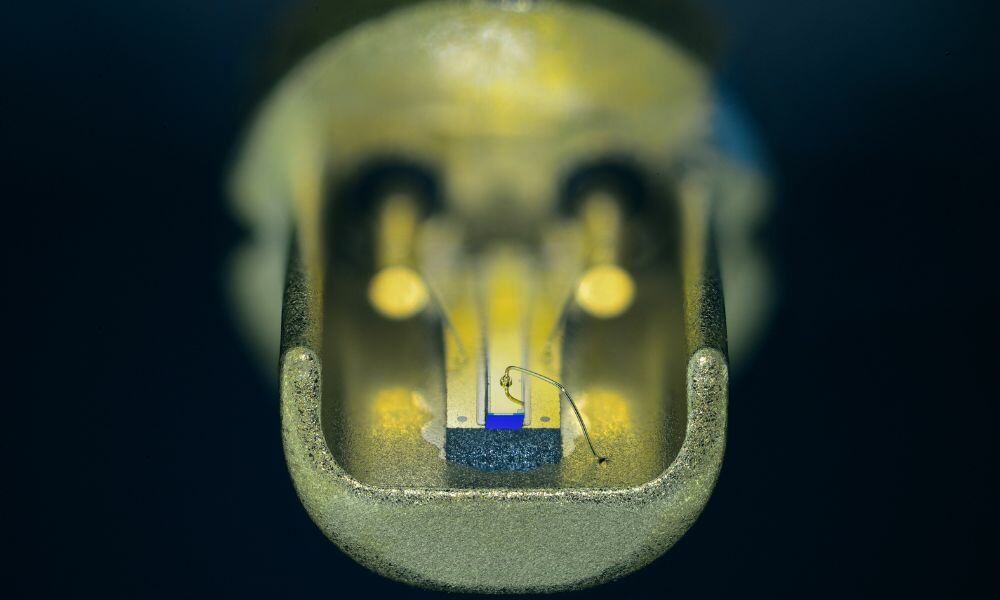This image features an intricate and abstract sculpture against a completely black background. The sculpture appears to be made out of a greenish-gray metal with pale green and blue accents, embodying the form of a skull. The lower part of the sculpture, which is distinctly U-shaped, almost like an upside-down arch, extends towards the foreground with a pale green hue, edged with darker green tones. This section vaguely resembles a wide-open mouth or jawline.

In the center of the sculpture, a thin wire extends upwards, then arches over and down, eventually touching the lower part of what can be interpreted as the mouth. The upper half of the sculpture is somewhat blurred, but it retains enough detail to hint at the shape of a skull, with eye sockets indicated by protruding gold cylinders and a nose section that stretches downward into a flat, rectangular form close to the mouth. The overall impression is of a large, electrified metallic skull sculpture, accentuated by its otherworldly green and gold tones against the stark black background.